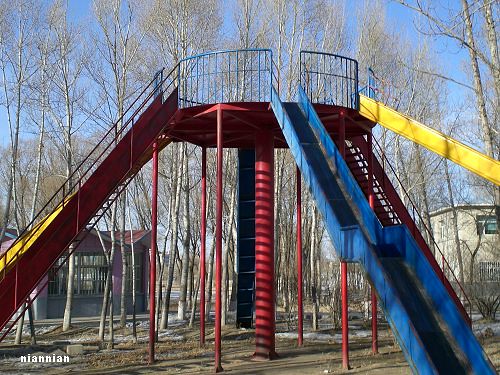In this photograph, taken during the daytime likely in autumn or winter, we see a towering, uniquely designed playground slide set situated in a park. This structure, primarily supported by a sturdy central red cylindrical pole and multiple smaller red metal poles, features a circular platform at its top, enclosed by blue safety railings. Extending from this high platform are four distinct slides, each diverging at different angles: a visible blue slide in the forefront with a metallic surface at the bottom, a yellow slide to the right, a red slide to the left, and a less distinct slide obscured behind. A set of red stairs on the right-hand side ascends from the ground to the platform, ensuring accessibility for children. The ground around the structure is noted to be dirt. In the bottom left corner of the image, the name "Nia Nian" is inscribed, potentially indicating the photographer. The backdrop includes several tall, leafless trees with slender white trunks, hinting at the season, and behind these trees, there are visible residential buildings, providing a peek into the surrounding neighborhood.